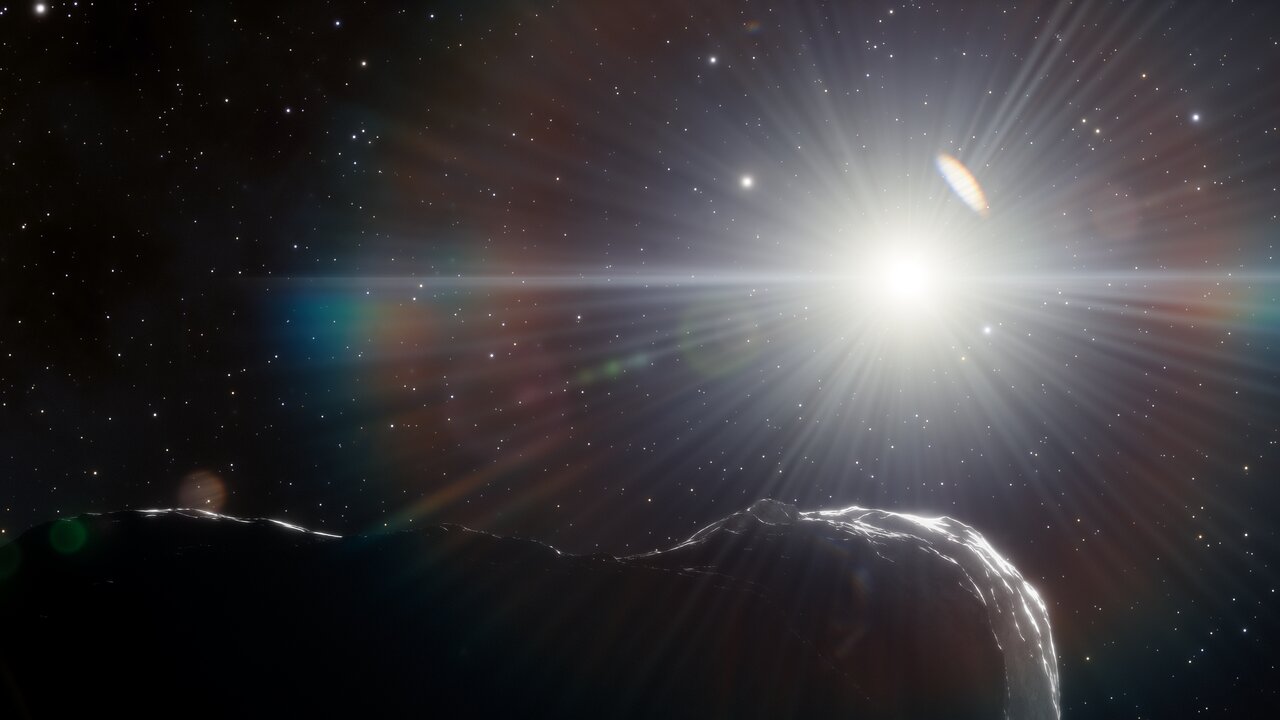In this captivating space image, a profound, dark sky forms the backdrop, speckled with countless twinkling stars of varying sizes. Dominating the scene, slightly off center to the right, is a radiant star with brilliant rays of light that cast a mesmerizing array of colors—shimmering blues, reds, yellows, and even hints of rainbow hues—across the cosmos. This star's dazzling light creates a vivid circle of color that contrasts starkly with the deep blackness beyond. In the foreground, prominently situated towards the bottom left, there looms a large, rocky mass, likely an asteroid, adding an element of mystery and grounding to the celestial panorama. The image, with its intricate interplay of light and shadow, leaves viewers pondering whether it's a genuine photograph from a space telescope or a skillful artistic rendition.